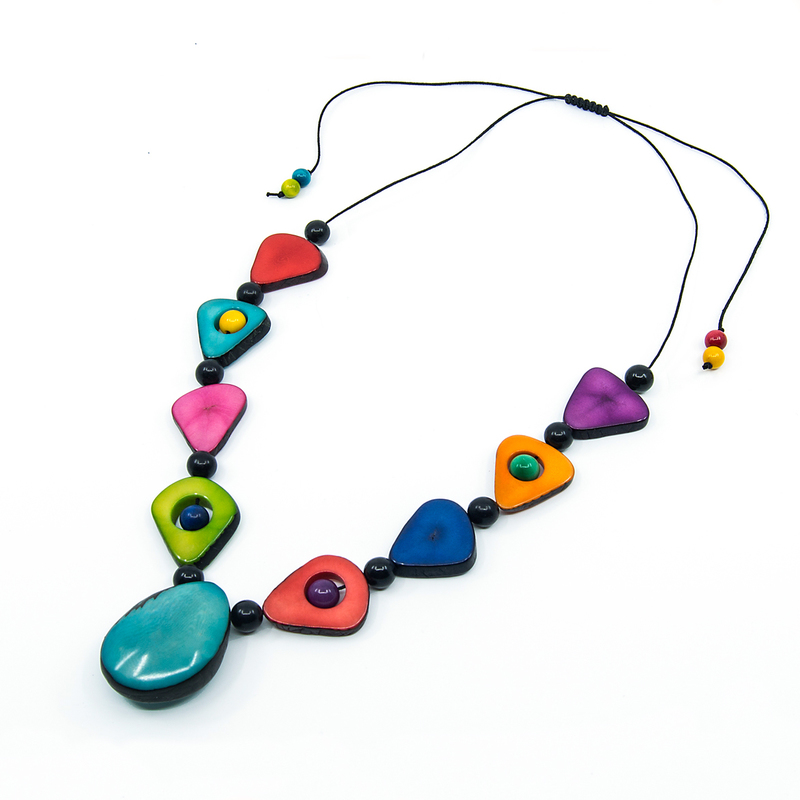This image showcases a meticulously designed necklace laid out on a white background. The necklace features a black cord adorned with a series of nine prominently positioned stones—eight triangular and one ovular. At the base of the necklace is a central, ovular, teal-colored stone, serving as the focal point. Flanking this centerpiece, on each side, are four triangular stones, separated by small, black spherical beads.

On the left side of the necklace, from bottom to top, the triangular stones consist of: 
1. A green stone with a blue bead in the center.
2. A pink stone.
3. A teal stone with a yellow bead in the center.
4. A red stone.

Conversely, the right side includes:
1. A red stone with a purple bead in the center.
2. A blue stone.
3. An orange stone with a green bead in the center.
4. A purple stone.

The necklace is knotted at the top, where two strings extend outward. The left string ends with a light green and blue bead, while the right string concludes with a red and yellow bead. The arrangement and color palette of the stones, alongside the meticulous details such as embedded beads, highlight the intricate craftsmanship of this accessory.